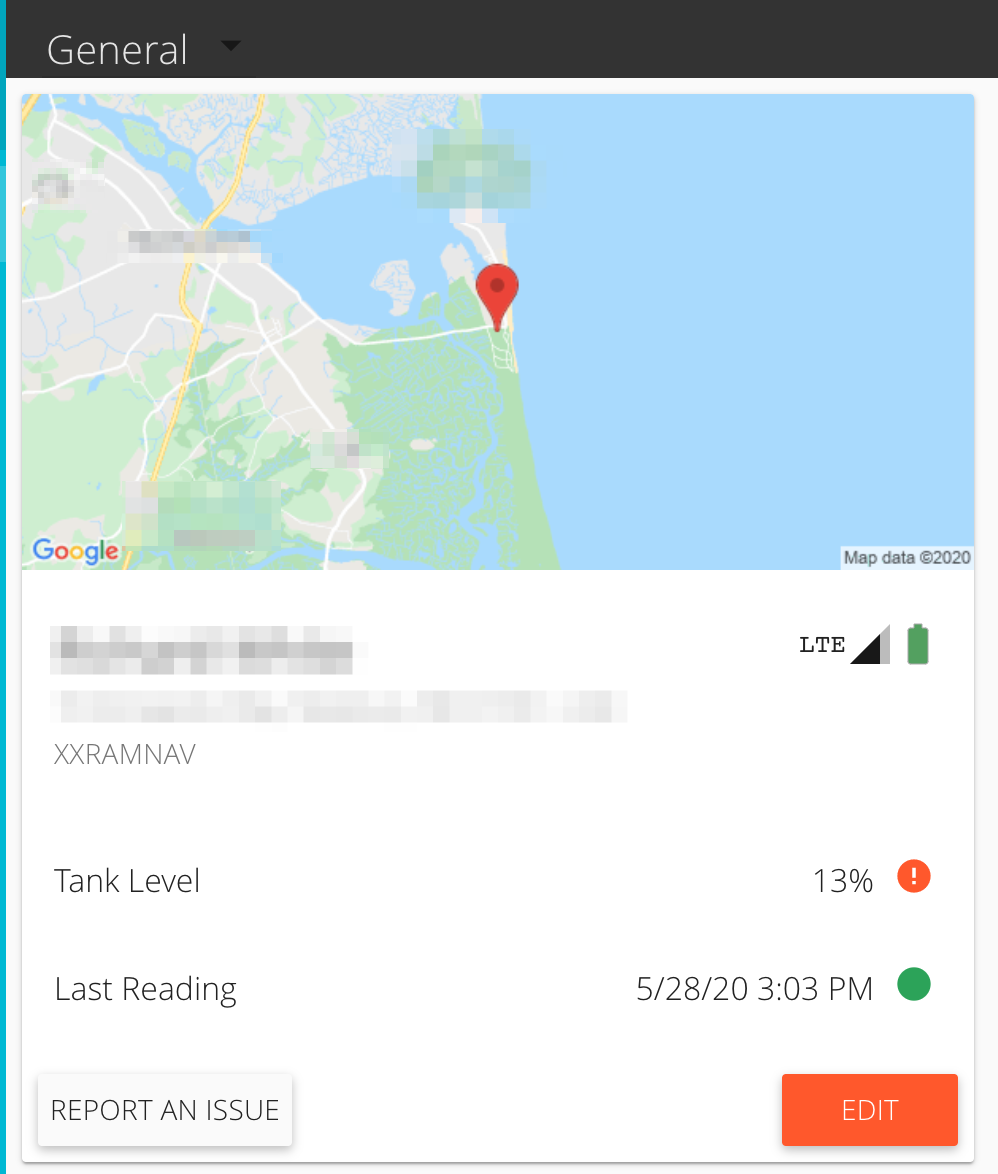This image is a screenshot of a user's phone displaying a partially censored Google Map with map data from 2020, likely showing a location on the eastern seaboard of the United States. The map reveals a significant amount of blue on the right side, suggesting the presence of the Atlantic Ocean or a major river. A red marker identifies the user's location near the coastline, amidst green areas indicating forested land. Rows of land or structures are visible in the map's layout.

At the top of the screen, a black bar with white text reads "General" on the top left, alongside a downward-pointing black arrow, suggesting a drop-down menu option. Beneath the map, text reads "XXRAM NAV," indicating that this may be from a navigation system, possibly within a vehicle. Additional information on the right side includes "LTE," the battery icon, and the signal strength indicator.

Further details note the vehicle’s tank level at 13%, accompanied by an orange exclamation mark, which serves as a warning. The last reading was taken on May 28, 2020, at 3:03 PM. Options to "Report an issue" and "Edit" are also present.